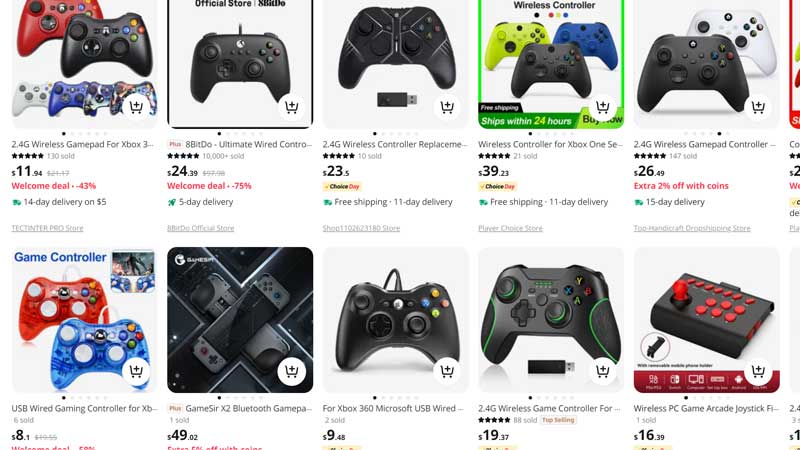A webpage displaying a catalog of wireless controllers for purchase is shown. The display consists of ten products organized in two rows, each featuring a variety of Xbox-formatted controllers. The controllers, predominantly black with some multicolored variations, come with different prices ranging from $8 to $49. 

In the top row, from left to right, the products are named:
1. 2.4G Wireless GamePad for Xbox 3, 
2. 8-bit DIL, 
3. Ultimate Wired Controller,
4. 2.4G Wireless Controller Replacement, 
5. Wireless Controller for Xbox One Series, 
6. 2.4G Wireless GamePad Controller.

In the bottom row, from left to right:
1. USB Wired Gaming Controller for Xbox,
2. GameSir X2 Bluetooth GamePad,
3. Microsoft USB Wired,
4. 2.4G Wireless GameController 4,
5. Wireless PC Game Arcade Joystick.

The majority of these products are handheld Xbox controllers, with a mixture of both wired and wireless options, and one arcade joystick.